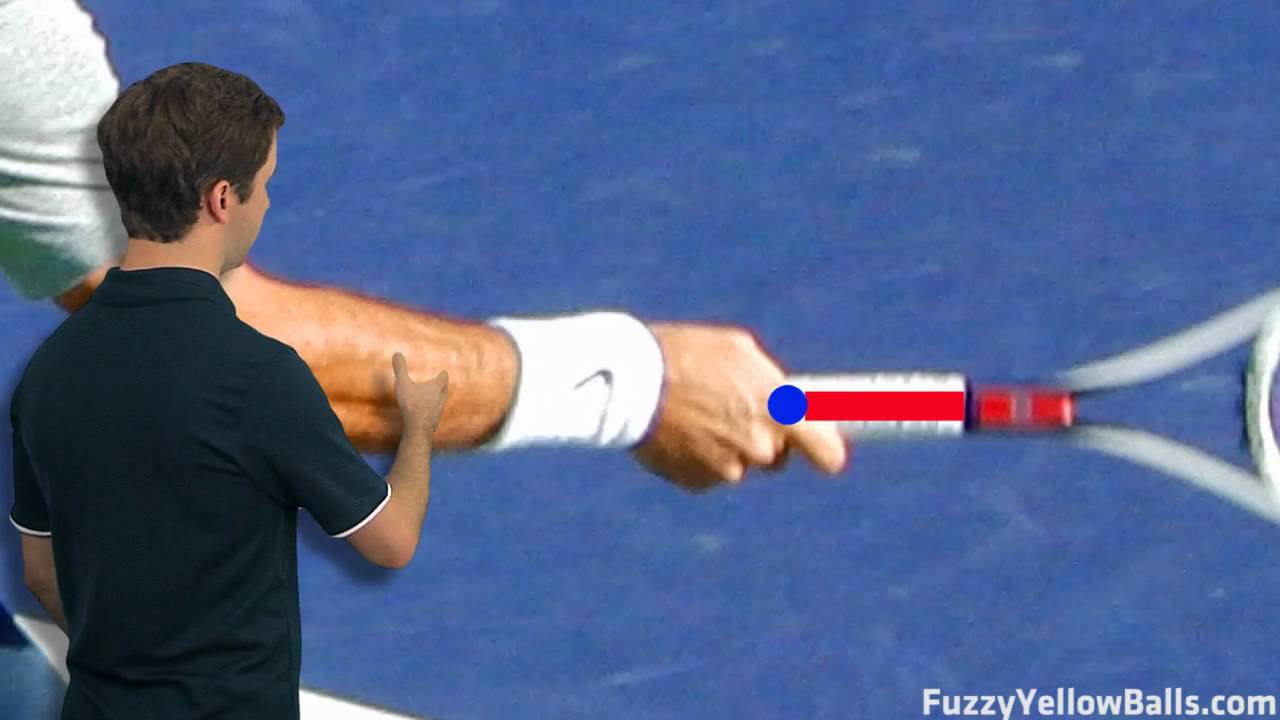This photograph features a white male with short brown hair, wearing a black t-shirt with white edges on the sleeves, gesturing towards a large screen TV. The screen displays a close-up of a tennis player's arm holding a racket, focusing on the mechanics of a tennis move. The tennis player is dressed in a gray shirt and a white wristband is visible on their arm. A computer graphic overlay consists of a blue dot and a red line, illustrating the movement and direction of the racket. The bottom right of the screen features the website fuzzyyellowballs.com in white font. The man is pointing specifically at the tennis player’s arm, emphasizing an essential aspect of the technique being demonstrated.